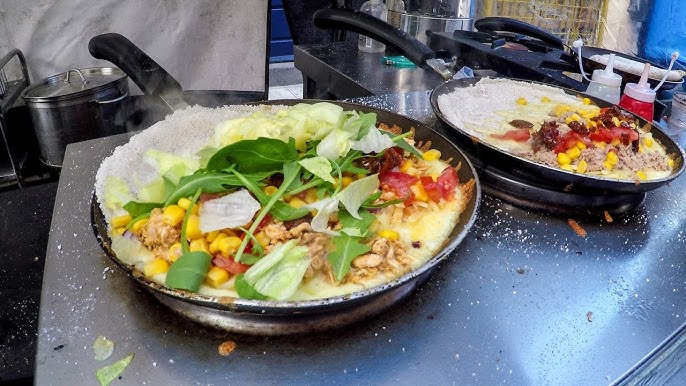In this industrial-style kitchen, a bustling scene features a large silver gallon pot in the background and a stainless steel cooking station in the foreground. Center stage are two sizable pans with black metal handles and stainless steel bottoms, both brimming with a colorful array of ingredients. The pan on the left appears laden with spinach leaves, arugula, chunky yellow pieces that resemble potato or corn, possibly some kind of meat, and vibrant red tomatoes or tomato chunks. Meanwhile, the pan on the right showcases yellow bits of corn, red tomatoes, fiery red chilies, and some ground meat. A messy stovetop suggests a lively cooking session, with crumbs scattered and two sauce bottles—one red and one clear—positioned to the far right. Overhead, stainless steel shelves and pots add to the industrious ambiance of the kitchen. This vibrant scene captures the making of a hearty breakfast, potentially a scrambled mixture or an omelet, full of fresh, colorful ingredients sizzling together.